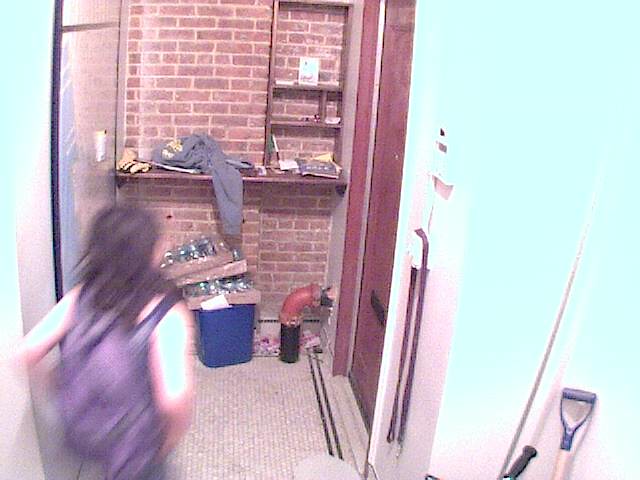In this image, a person wearing overalls, a white shirt, and with long black hair is seen walking into a room. The individual is captured from behind. On the right-hand side, the top handles of several shovels are visible, identifiable by their distinctive shapes. The room features a light blue wall that gradually becomes lighter towards the base. To the left of the shovels, there is a brownish-red door framed by a matching frame. In the background, a brick wall is partially visible, adorned with a brown shelving unit on the right and an additional shelf beneath it. Various cardboard boxes are stacked on these shelves, and a red pipe emerges from the wall above. The floor is covered in gray bathroom tiles, and to the left of the image, there is a clear window with a black outer frame.